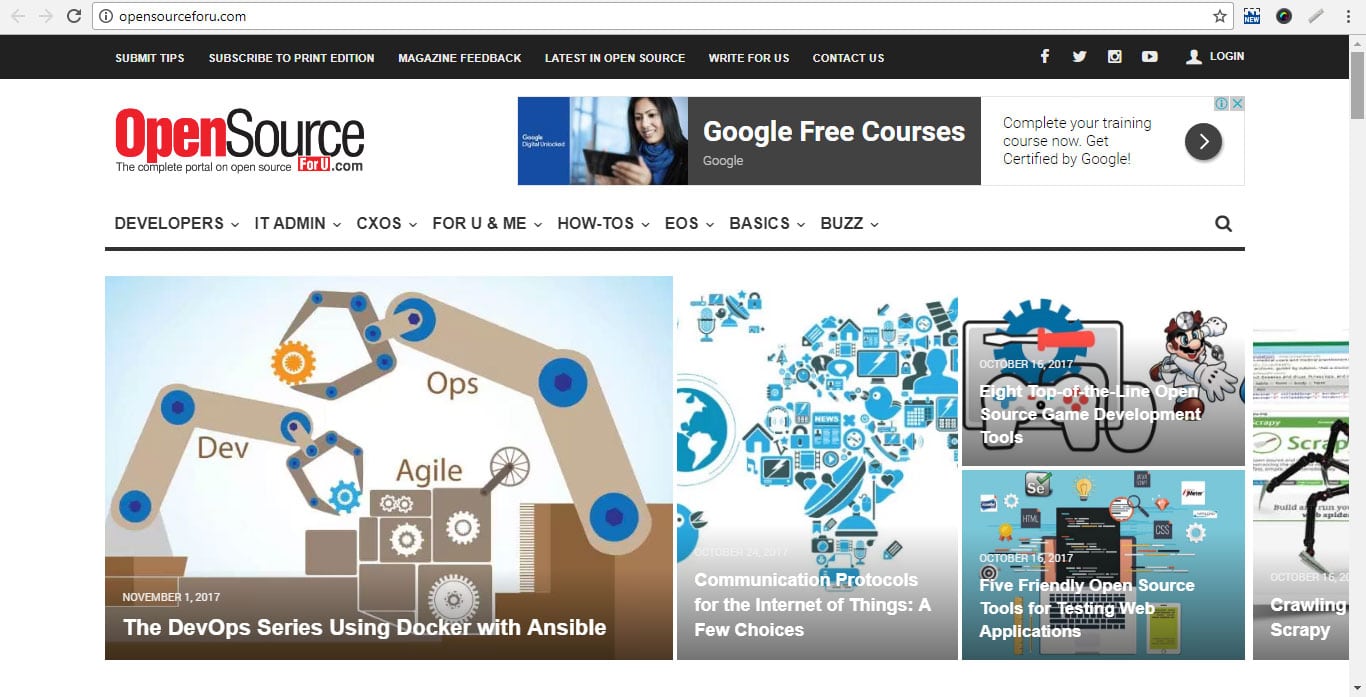At the top of the image, on the left side, is a refresh icon, and on the right, there are four additional small icons. Below this section is a black background featuring six categories written in very small white text. Adjacent to this, on the right, are icons representing four major social media platforms—Facebook, Twitter, Instagram, and YouTube—with a white login option further to the right.

Beneath this area, the text "open source" is displayed, with "open" in red and "source" in black. To the right of this, there is an advertisement for Google's free courses. Below this section, categories are listed from left to right, including Developers, IT Admin, CXOs, For You and Me, How To, EOS Basics, and Buzz.

In the next section, five main options are displayed. The largest option on the left highlights "The DevOps Series: Using Docker with Ansible" and includes a corresponding diagram. To the right of this, there is an option titled "Communication Protocols for the Internet of Things," featuring a diagram of several countries and continents in blue. Adjacent to this are two options stacked vertically, with the top option placed above another. To the extreme right, the content appears to be partially cut off, and the text "crawling and scrappy" is visible at the bottom. A scrollbar is situated on the far right side of the page, indicating that the user is currently at the top of the page.